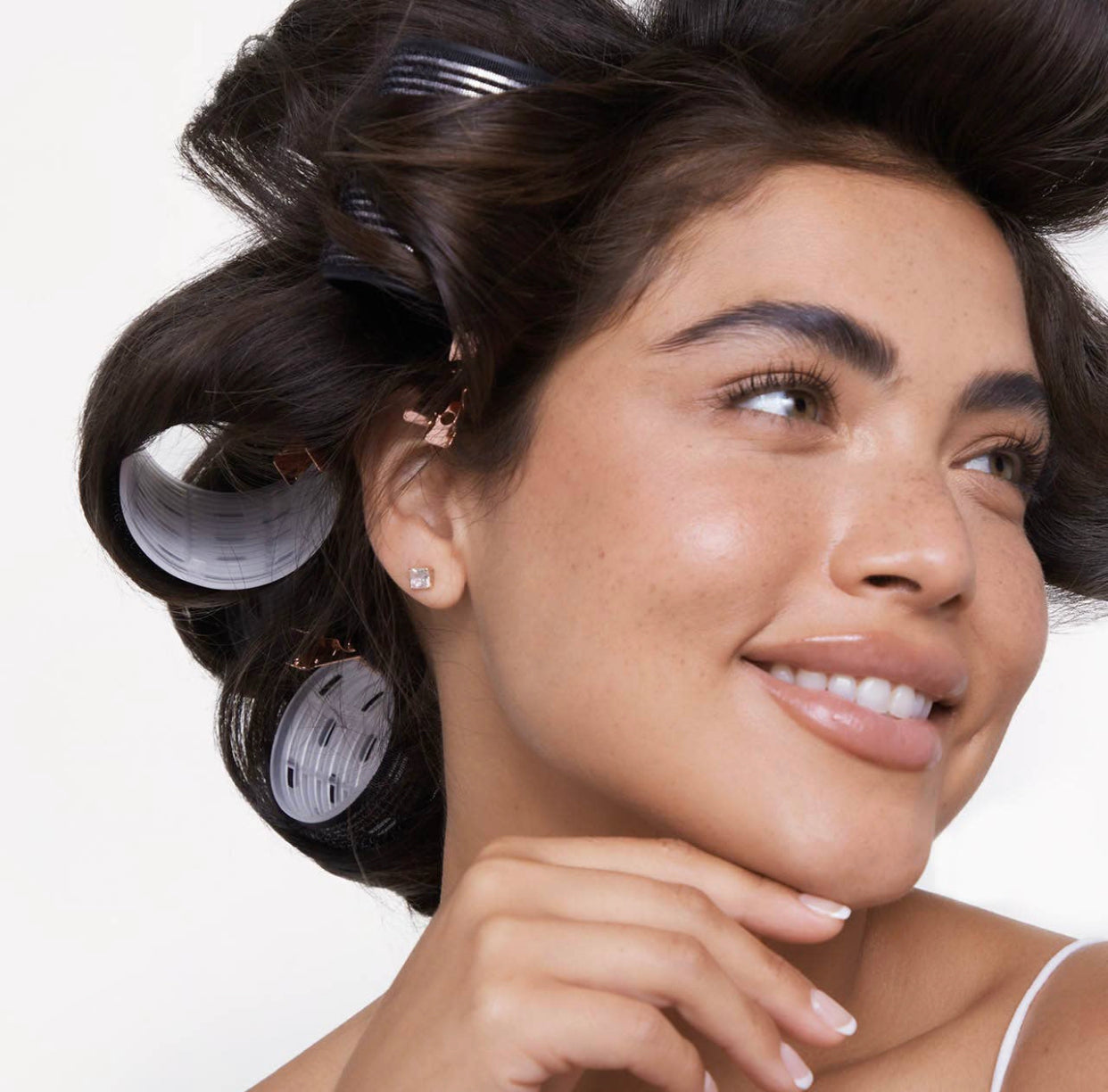This is a full-color, vertically rectangular photograph, likely taken indoors with artificial lighting by a professional photographer. The background is a light gray, providing a neutral setting that draws attention to the subject— a young, light-skinned Black woman with a beautiful, healthy appearance. She is smiling, revealing her perfect white teeth, and her hazel eyes are looking off to the right side of the image. Her hair, long and straight, is styled with several large, white plastic curlers, two or three of which are visible. 

The woman's attire includes a white spaghetti strap top visible over one shoulder. Her right hand, positioned gracefully under her chin, reveals four well-manicured fingers and polished nails. Additionally, a small, diamond-like stud earring adorns her right ear, adding a touch of elegance to her poised and serene expression.